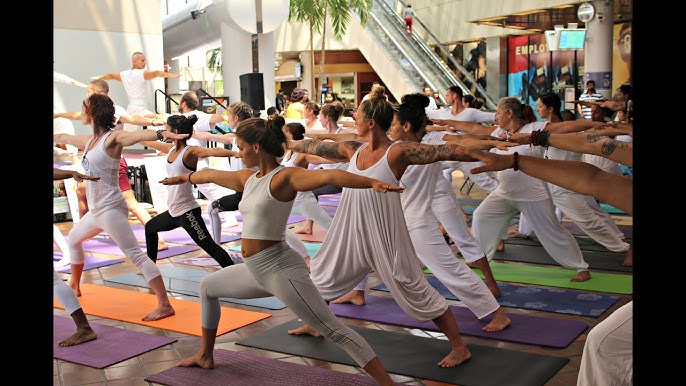The photograph depicts a unique and intriguing scene of a large group of people participating in a yoga session inside what appears to be a shopping mall. The setting combines elements of both fitness and retail environments, creating an unusual but captivating image. In the foreground, numerous individuals dressed mostly in white workout attire perform uniform yoga poses on colorful mats scattered across the floor. Among them is a notable exception, a woman in black pants branded with "Reebok." 

The yoga practitioners are facing towards the left, where a stage is positioned. On the stage, there are two individuals who appear to be instructors guiding the session. The backdrop of the image reveals typical mall features, including a building with an escalator and several stores. Further adding to the realism and everyday nature of the scene, there are small trees in the mall area and a person visible mid-ascent on the escalator. The juxtaposition of a serene yoga practice within the bustling environment of a shopping mall makes this photograph both striking and memorable.